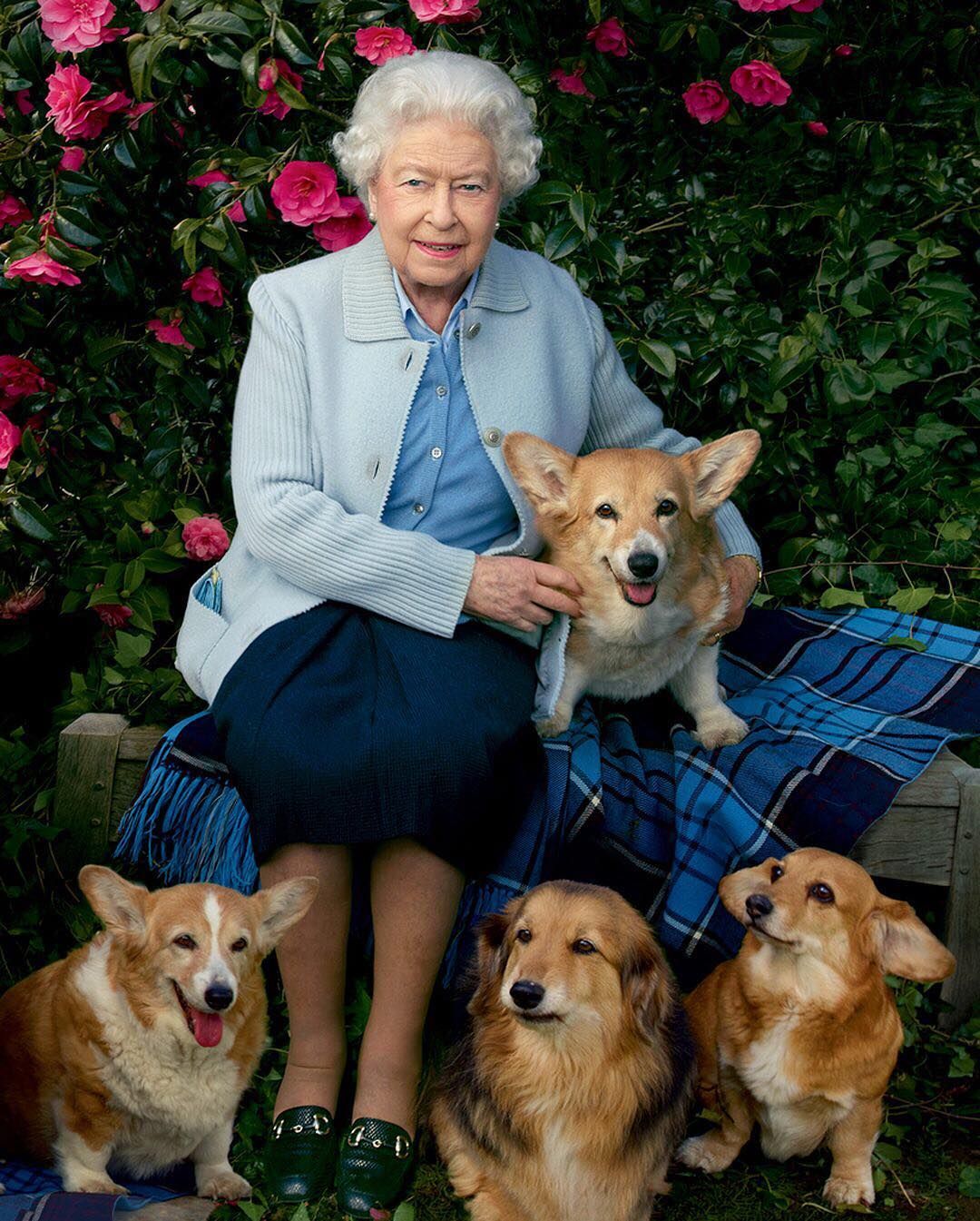A photograph captures an older Queen Elizabeth II sitting serenely on a stone bench, adorned with a blue and black plaid Afghan blanket with fringes. Her silvery hair frames her serene face, where she smiles gently, accentuated by her signature lipstick. She is dressed in a light blue cardigan over a slightly darker blue button-up shirt, paired with a dark navy skirt that falls just below her knees, and black shoes. In her right pocket, there appears to be a small item. The Queen is accompanied by her beloved corgis: three at her feet and one nestled by her side on the blanket. The corgis, mostly beige and white, gaze towards the camera, with one appearing to be a mix or possibly a long-haired corgi. Behind her, a lush rose garden in full bloom showcases deep, pinkish-red roses against dark green foliage, adding a vibrant and nostalgic backdrop to this touching family portrait. The setting is outdoors, invoking a sense of peaceful, royal leisure.